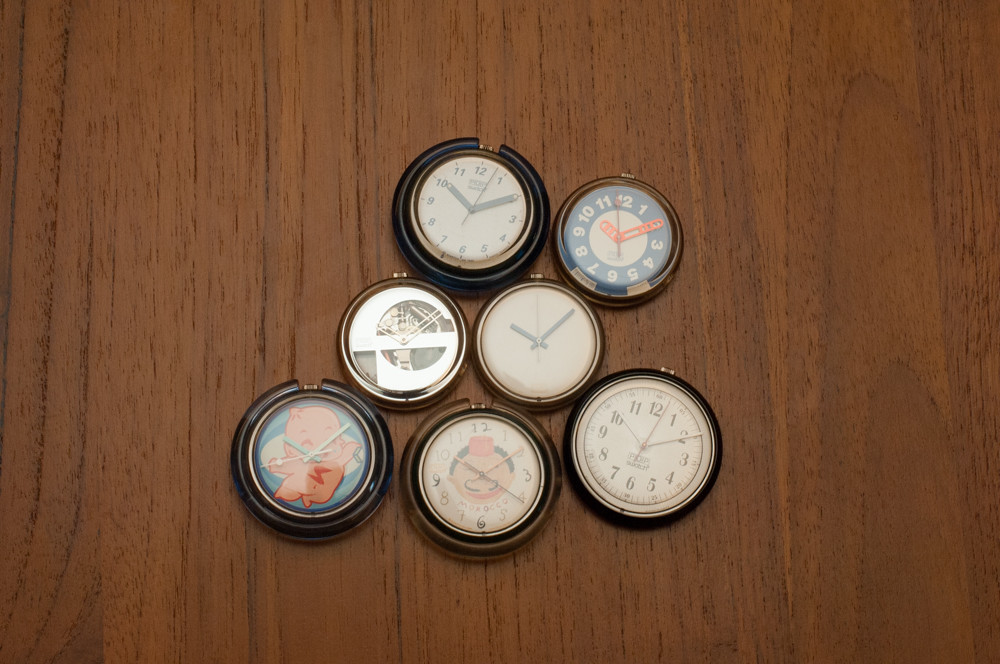The photograph features a close-up top-down shot of seven vintage analog watches arranged on a dark chocolate brown wooden table. Each watch has a circular face, varying in designs and colors, accentuating their uniqueness. The upper-left watch sports a white face with a black rim. To its right, a distinctive blue face with red hands stands out, showing the time at 10:10. The center watch is framed in gold with a white face and black hands, also reading 10:10. 

Moving to the lower-left, there's a charming retro watch with a baby doll illustration against a blue backdrop, detailed with light blue hands. The center watch below features a cartoon-like man with black hair, gold hands, and a brown rim. Notably, one watch displays the intricate inner mechanism through a gold cutout 'S' shape, offering a glimpse into its workings.

Lastly, the bottom-left showcases a delicate clock with a joyful cherub set against a sky blue background, exuding a whimsical vintage charm. While several of the watches retain traditional numeric markings from 1 to 12, others emphasize minimalist design, foregoing numbers entirely. Each watch is adorned with a top button, indicative of classic stopwatch functionality, blending artistry with old-fashioned craftsmanship.